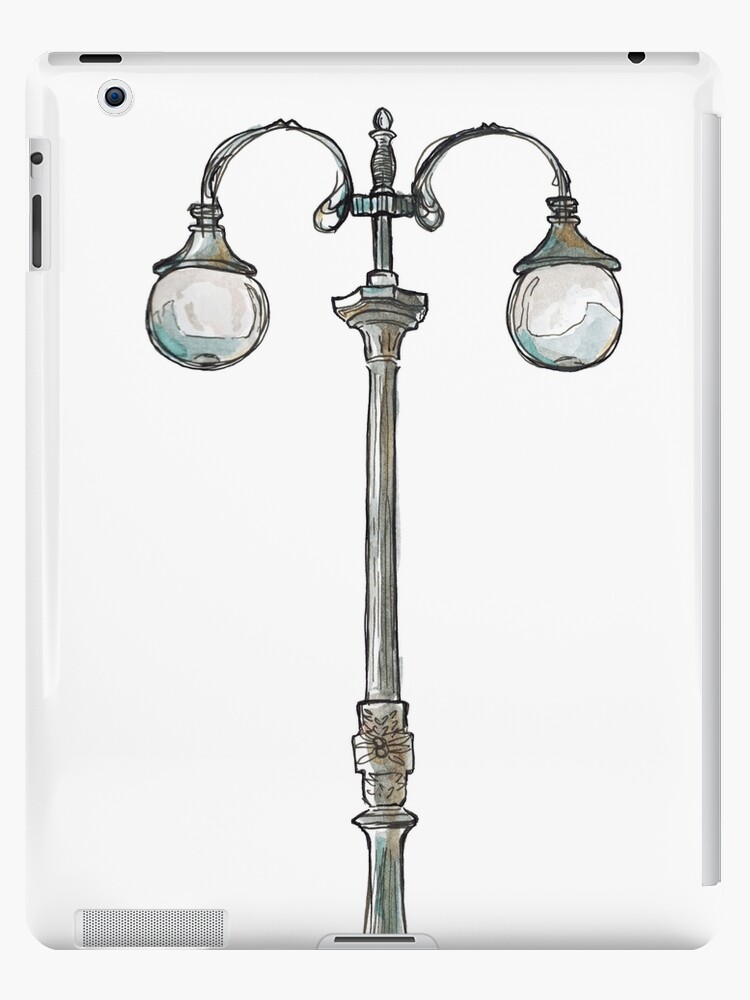The image is an illustration of a tall, intricately designed streetlamp set against a white background. The lamp features a central pole, which appears to be made of iron or metal, adorned with black and light blue lines and a light brown pattern in the middle. The base has a rounded white section with a black-etched flower design. Moving upward, the pole is crowned with a star-shaped finial connected to a rounded top edge. The lamp has curved arms that extend to the left and right, each ending in cone-shaped mounts that hold globe-shaped lamps. These lamps are clear, with white and light blue teal sections underneath. The entire illustration seems to be a decorative design on the back of a tablet cover, likely an iPad, indicated by the presence of multiple small holes and vents for the device's functionalities. The cover appears to be white, with sections for a camera lens, headphone jack, and additional ports.